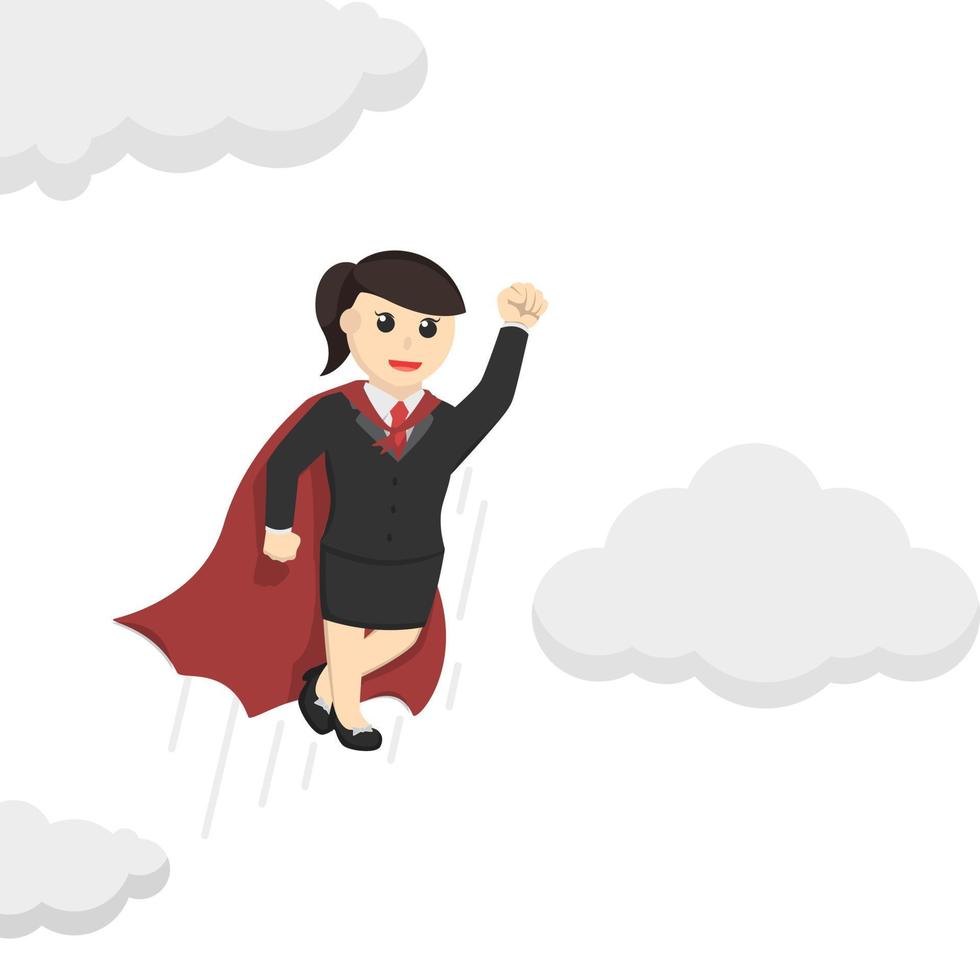This cartoon digital illustration, rendered in a simple corporate clip art style, features a Caucasian woman with dark brown hair pulled back into a ponytail, embodying a superhero persona. She is dressed in a formal attire that resembles a school uniform: a black blazer paired with a white shirt and a red tie, complemented by a black skirt and black shoes. A striking red cape is tied around her neck, fluttering behind her as she assumes a dynamic pose with her left fist raised and her right hand at her side, suggesting she is flying.

The background is a stark white void, accentuated with three gray clouds: one fully visible cloud to her right, another large fluffy cloud in the top left corner, and a partial cloud at the bottom left. Action marks around her give the impression of flight, enhancing the scene's energetic and whimsical atmosphere.